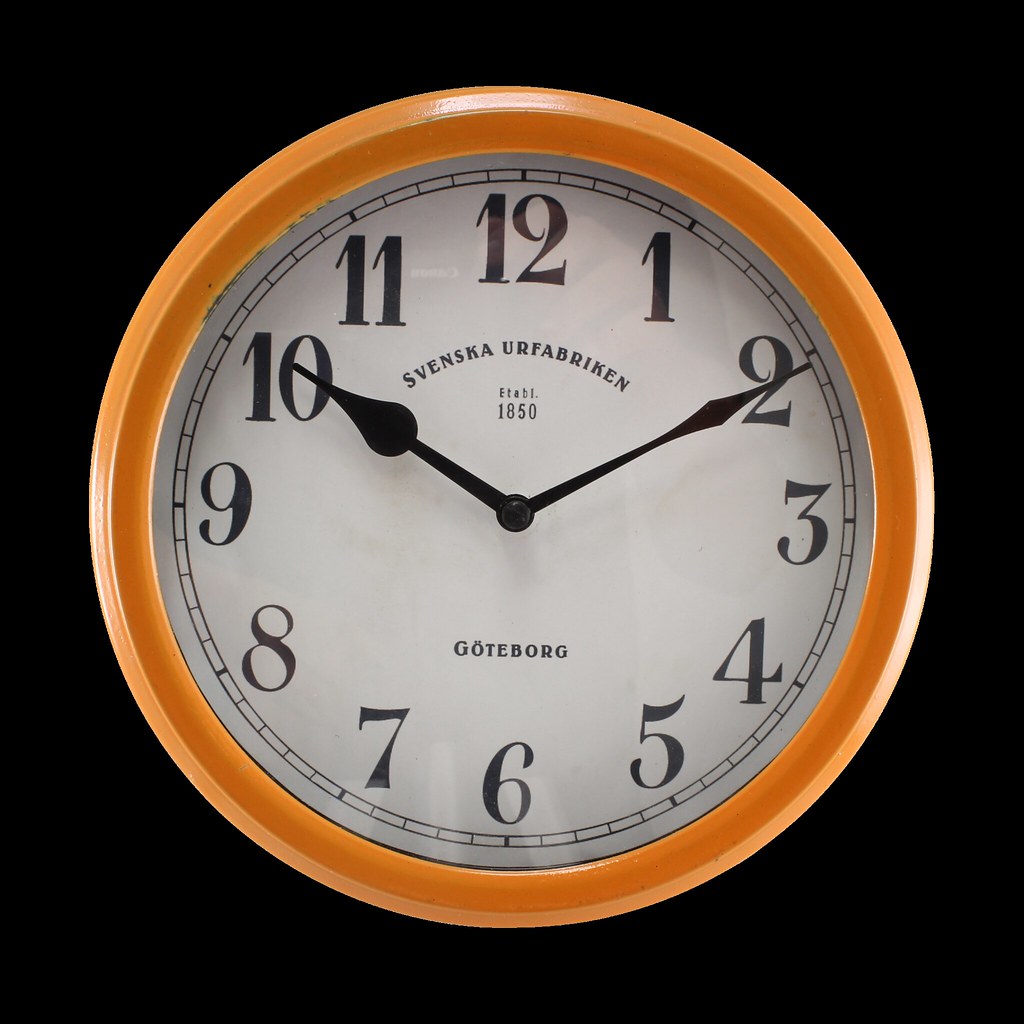The image showcases a clock positioned against a black square background. The clock is circular in shape and features a vibrant orange outer rim. The dial of the clock displays the numbers 1 through 12, all written in bold black font. The clock's hands are also black, providing a striking contrast against the orange and white face. 

Notably, there is an inscription at the center of the clock face. The top part of the inscription reads "SVENSKA URFABRIKEN," which appears to be the manufacturer's name, though it is not widely familiar. Below this, the clock states "Est. 1850," indicating its establishment year. Further down, just above the 6 o'clock position, the text "GÖTEBORG" is prominently displayed in all capital letters, with two dots accentuating the 'O' in true Swedish orthographic tradition. All these details contribute to a detailed and vintage aesthetic of the clock.